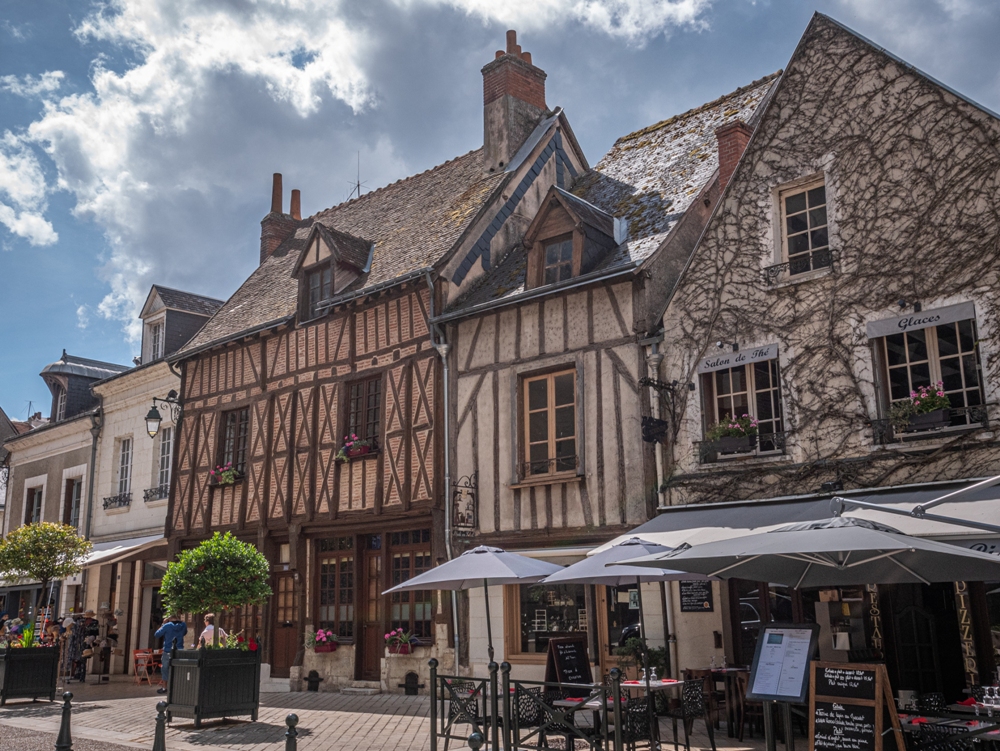The image depicts a charming old commercial street, possibly in a European village, lined with a series of narrow, two-story buildings of varying heights and decorations, all forming a continuous facade. Central to the scene, two buildings embody the Tudor half-timber style with visible wooden beams arranged in X-shaped patterns. Flanking this architectural ensemble is a gray stone building on the right, entirely cloaked in ivy, contributing to the historical medieval ambiance. In front of this ivy-clad structure and stretching along the entire row is a brick plaza, adorned with tables and umbrellas typical of outdoor café seating. A chalkboard menu stands invitingly outside the ivy-covered building, while trees and portable wooden cubicle pots punctuate the plaza, further enhancing the picturesque, old-world charm of the scene.